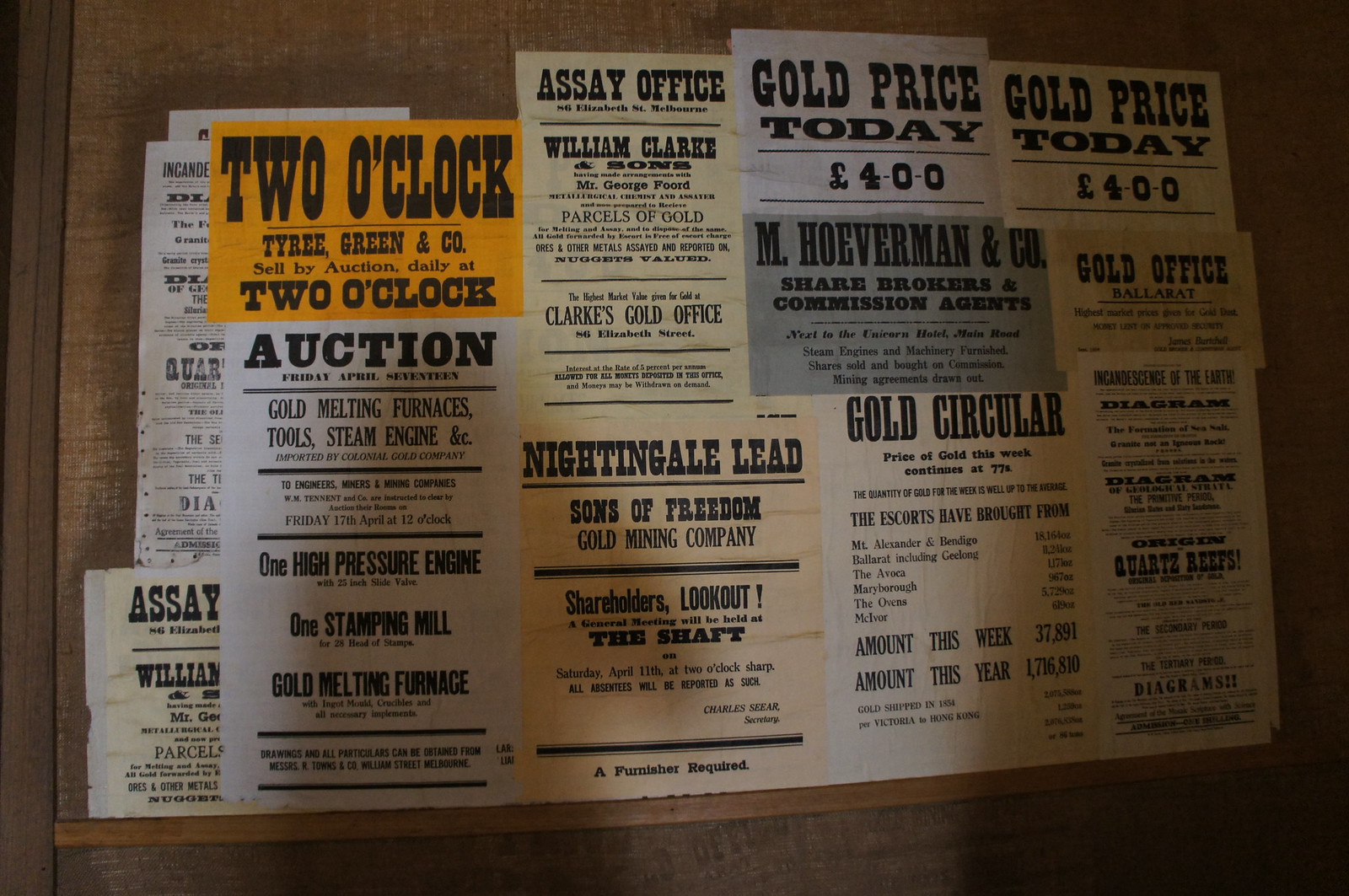This detailed image depicts a cork board covered with various colorful flyers and advertisements, primarily focused on gold auctions and mining enterprises, reminiscent of an old-time western town. Dominating the board are papers in colors like yellow, cream, white, gray, and shades of orange. Notably, a bright yellow paper announces "Tyree Green and Company sell by auction daily at 2 o'clock," underscoring the daily auction time. Another significant flyer in black print on a white background lists items such as "gold melting furnaces, tool steam engine, one high-pressure engine, one stamping mill." A tan flyer advertises an "assay office by William Clark and Sons," and there are multiple mentions of "Nightingale Lead, Sons of Freedom, Gold Mining Company." Across the board, other flyers highlight gold prices, such as "gold price today is $4," and several posters bear the name "M. Hoverman and Company, share brokers and commission agents." The composition of these flyers suggests a historical setting focused on gold trading and auctions, capturing a fragment of bustling commercial activity in a bygone era.